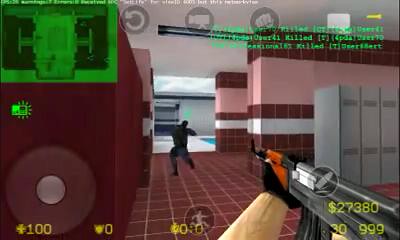This is a detailed screenshot from a first-person shooter game. In the lower right corner, the player’s white character arm, clad in black gloves, is gripping the front end of a futuristic firearm that features a color palette of gray, red, and white. The gun is aimed at a mysterious black figure located in the center of the image, which is walking on a floor paved with red tiles. Surrounding the scene, the walls are adorned with a combination of red tiles, pink paint, and white tiles.

The black figure appears to be moving towards the back of the room, where the floor transitions into white and blue tiles, possibly leading to an area with a gray window or screen. On the right side of the image, there are several gray lockers lined up. Near the bottom of the screen, there are various numerical statistics displayed: "100", "0", "0", and "$27,380 / $30,999." At the very top of the image, there is a green banner with text, accompanied by icons including a return arrow, a camera, and a fist symbol, providing additional user interface elements for gameplay. 

Overall, the scene suggests an intense and tactical environment, depicting a moment of potential confrontation within a vividly detailed game world.